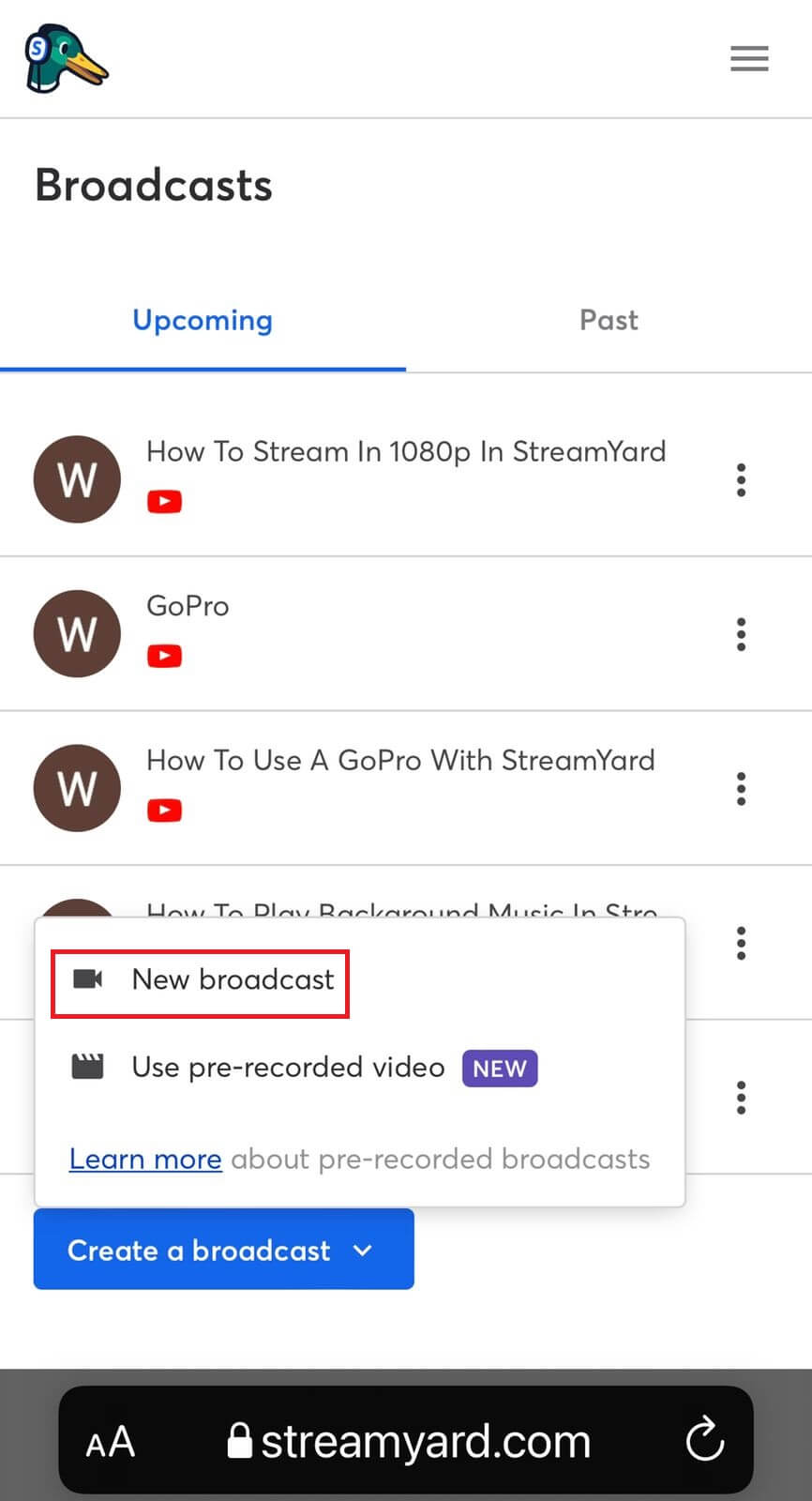The image depicts a cell phone application interface, likely belonging to StreamYard, an online broadcast tool. 

### Upper Section:
- **Icon**: On the upper left, there is a distinctive duck wearing headphones icon with an 'S' in the middle.
- **Label**: Directly beneath the duck icon is the word "Broadcast".

### Tabs:
- **Upcoming**: A blue highlighted tab labeled "Upcoming".
- **Past**: A tab labeled "Past" next to the "Upcoming" tab.

### Body Section:
- **Title**: The primary title displayed is "How to Stream in 1080p in StreamYard".
- **Subtitles and Icons**:
  - Below the main title, there is the Google Play icon followed by the word "GoPro".
  - Further down, the YouTube icon appears with the subtitle "How to use a GoPro with StreamYard".

### Overlay Popup:
- **Popup Description**: A pop-up dialog partially obscures the content, presenting options "New Broadcast" or "Use Pre-recorded Video".
- **New Badge**: A small box labeled "New" in purple or blue.
- **Learn More**: Below the popup, there is a link stating "Learn more about prerecorded broadcasts".

### Action Buttons:
- **Create Broadcast**: A prominent blue button labeled "Create a Broadcast" with a downward-facing arrow.

### Bottom Section:
- **Search and Website Indicator**: At the bottom, an icon indicates StreamYard.com, accompanied by a lock icon to denote a secure site.
- **Background**: The predominant background is white, but at the very bottom, there is a black bar featuring the StreamYard.com label against a slight gray backdrop.

Overall, the interface is straightforward, with a focus on providing options for broadcasting and learning about streaming techniques.